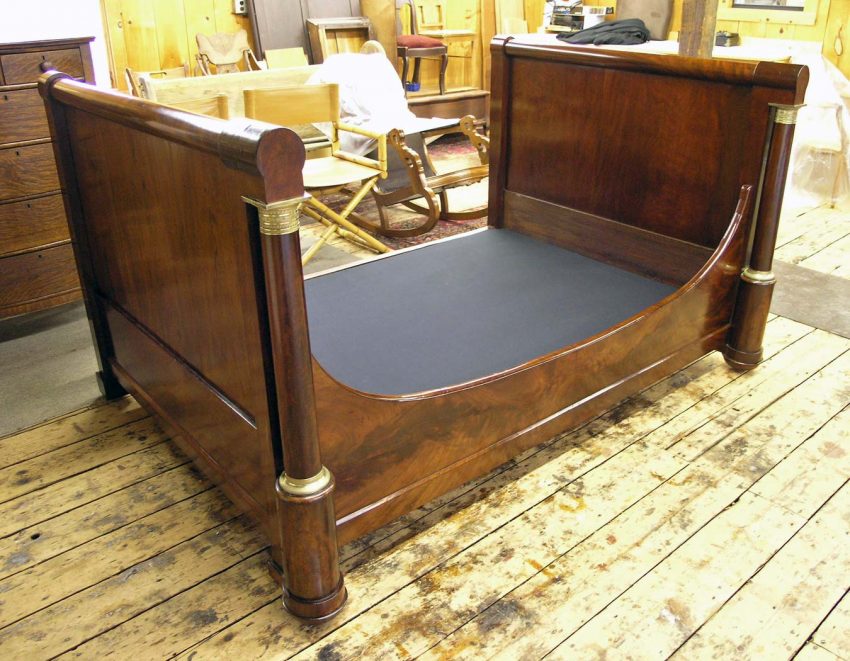The image showcases a rich, dark brown wooden bed frame without a mattress, beautifully highlighted by its polished finish and accented with gold trim. The bed, which hints at a sleigh style with an inverted arch on the near side, rests on weathered, beige wooden floorboards marred by dark brown patches and signs of rust or weather damage. To the left of the bed, there is a matching dresser and a rattan rocking chair draped with a white blanket. Additionally, two director's chairs, typically seen on a movie set, are present. The background features various other pieces of furniture. The room itself has wooden walls, constructed from newer, unfinished cabin wood, which doesn't quite match the rustic barn floor. Near the window, which is partly out of the frame, stands a red stool, adding a splash of color to the otherwise earthy-toned space.